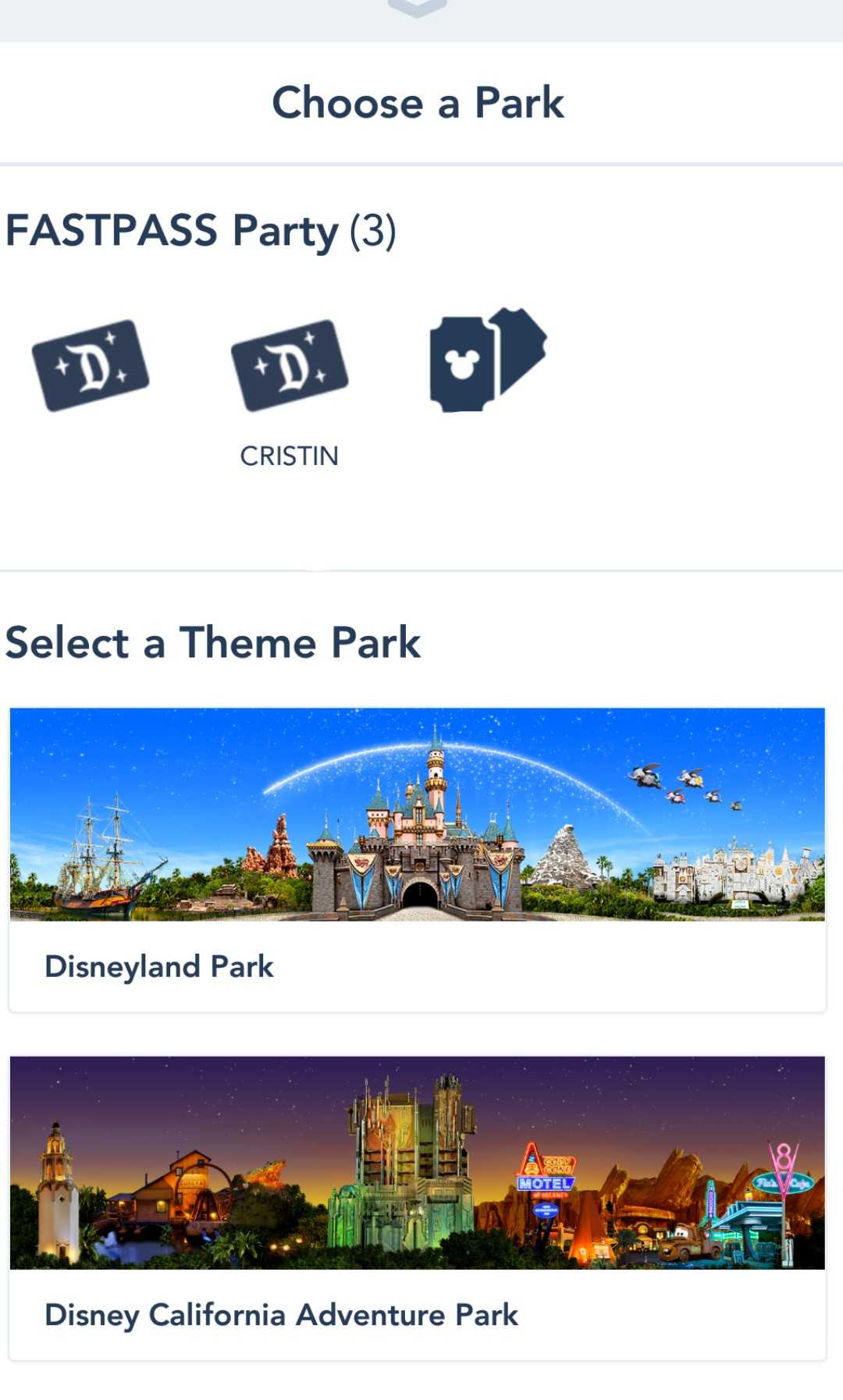This detailed digital image captures the vibrant essence of theme parks, prominently featuring Disneyland and Disney California Adventure Park. At the top, the interface presents an option to "Choose a Park," accompanied by a "Fast Pass Party" indicator with the number three in parentheses. Additionally, the name "Kristen" is displayed alongside a recognizable Mickey Mouse logo. Following this, two stylized D's surrounded by stars frame the prompt to "Select a Theme Park."

The image includes a colorful, animated depiction of Disneyland, highlighted by iconic elements such as flying elephants from the Dumbo ride, a magnificent large castle, lush palm trees, and a pirate ship. Just below, Disney California Adventure Park is introduced with a striking image of a white and gold lighthouse, more palm trees, another grand castle, a quaint motel, and an animated truck, creating a whimsical and inviting scene for viewers.